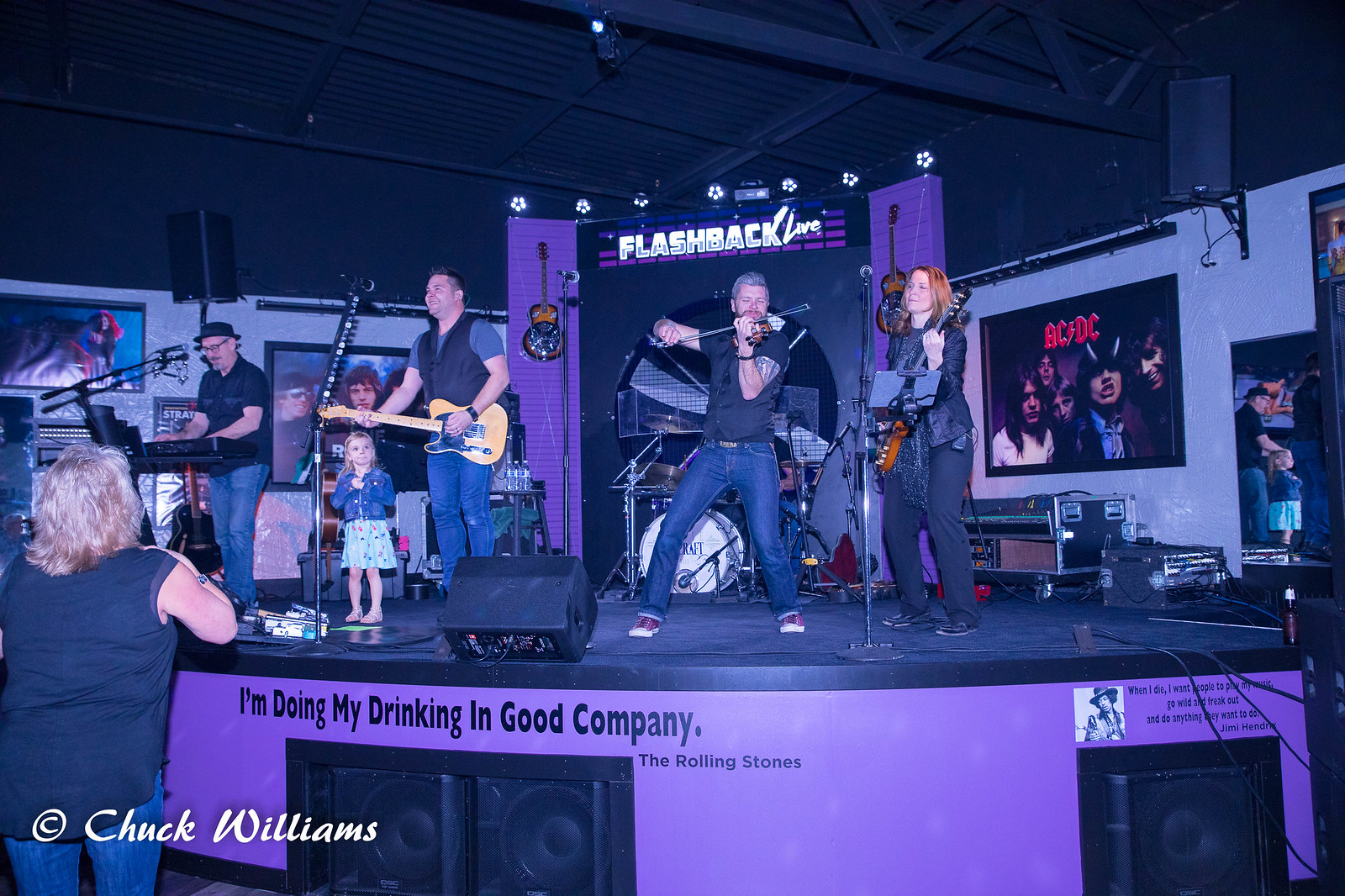The photograph captures a dynamic scene of a band performing on a stage inside a bar. The stage, predominantly black with a purple front, is set with black speakers. A man with gray hair, centered in the image, passionately plays a violin or fiddle, clad in a black shirt and blue jeans. To his left, a man wearing a blue shirt under a black vest, paired with blue jeans, is engaged with a bass or guitar. Further left, a small blonde child in a blue jean jacket and skirt stands curiously near the musicians. A man on keyboards, donning a black hat, black shirt, and blue jeans, is seen next to her. On the far right, a woman with long brown hair, dressed entirely in black, strums a bass or guitar.

The backdrop features grayish walls with a large black centerpiece bordered in purple, emblazoned with “Flashback Live” in white text against the purple. A drum set remains partially hidden behind the central violinist. The stage's front displays the phrase “I’m doing my drinking in good company, The Rolling Stones” in black text across the purple surface. Below the stage, a woman with short blonde hair, wearing a sleeveless black shirt and jeans, leans casually, absorbing the performance. The walls behind are adorned with band photos, including one of AC/DC on the right side. At the bottom left corner of the image, the text “See Chuck Williams” can be faintly observed, adding a touch of personal significance to the scene.